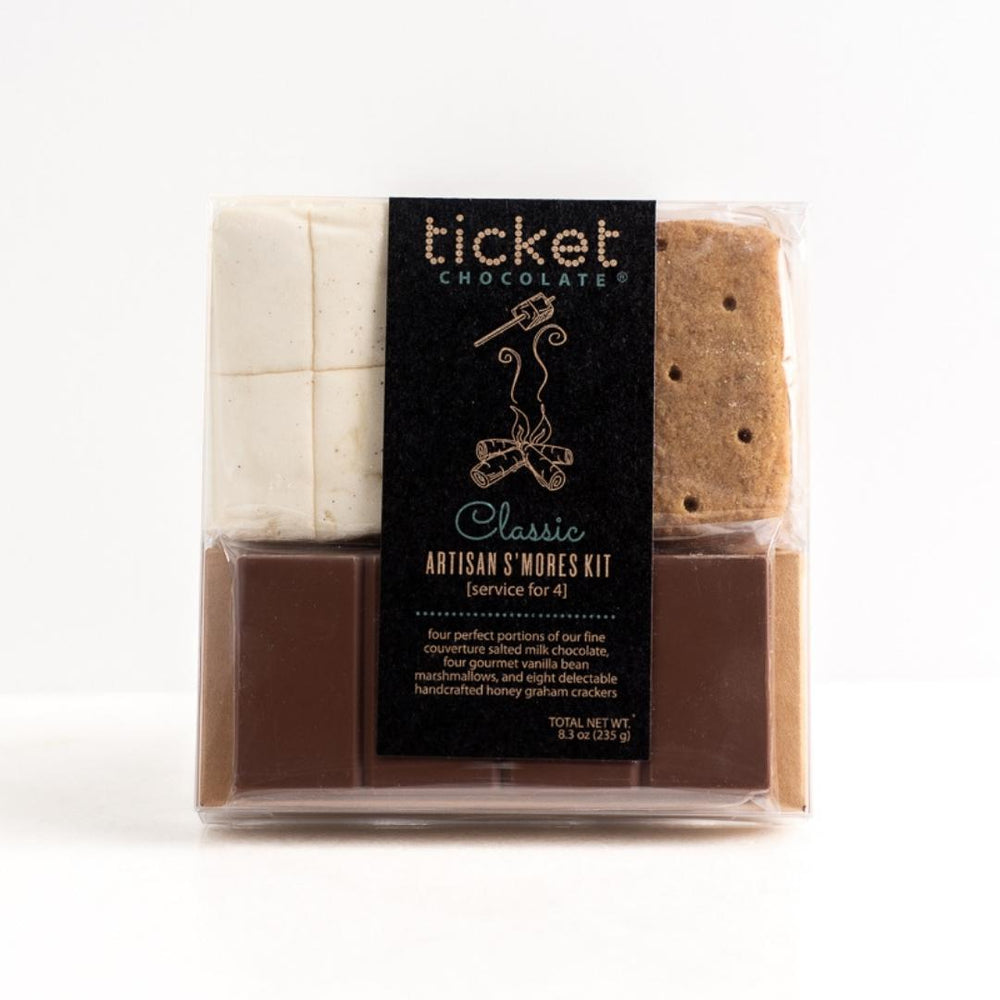The image depicts a Ticket Chocolate Classic Artisan S'mores Kit, neatly arranged on a white background. The entire kit is wrapped in clear plastic, secured with a sophisticated black label adorned with gold text. At the top, the label features the gold word "TICKET," followed by "CHOCOLATE" in gray. Below this, a gold-outlined drawing of a campfire with a marshmallow on a stick sets a cozy scene. In dark gray, it reads "CLASSIC," and further down, in gold, "ARTISAN S'MORES KIT, service for four."

This kit promises four perfect portions of their fine salted milk chocolate, four gourmet vanilla bean marshmallows, and eight delectable handcrafted honey graham crackers, with a total net weight of 8.3 ounces. The items are strategically arranged inside the package for convenience: the marshmallows are at the top, the chocolate bars are at the bottom, and the graham crackers are on the right. The marshmallows appear larger and longer than typical ones, potentially needing to be cut. This thoughtfully packaged kit contains all the essentials to create four sumptuous s'mores, showcasing an emphasis on quality, convenience, and artisanal craftsmanship.